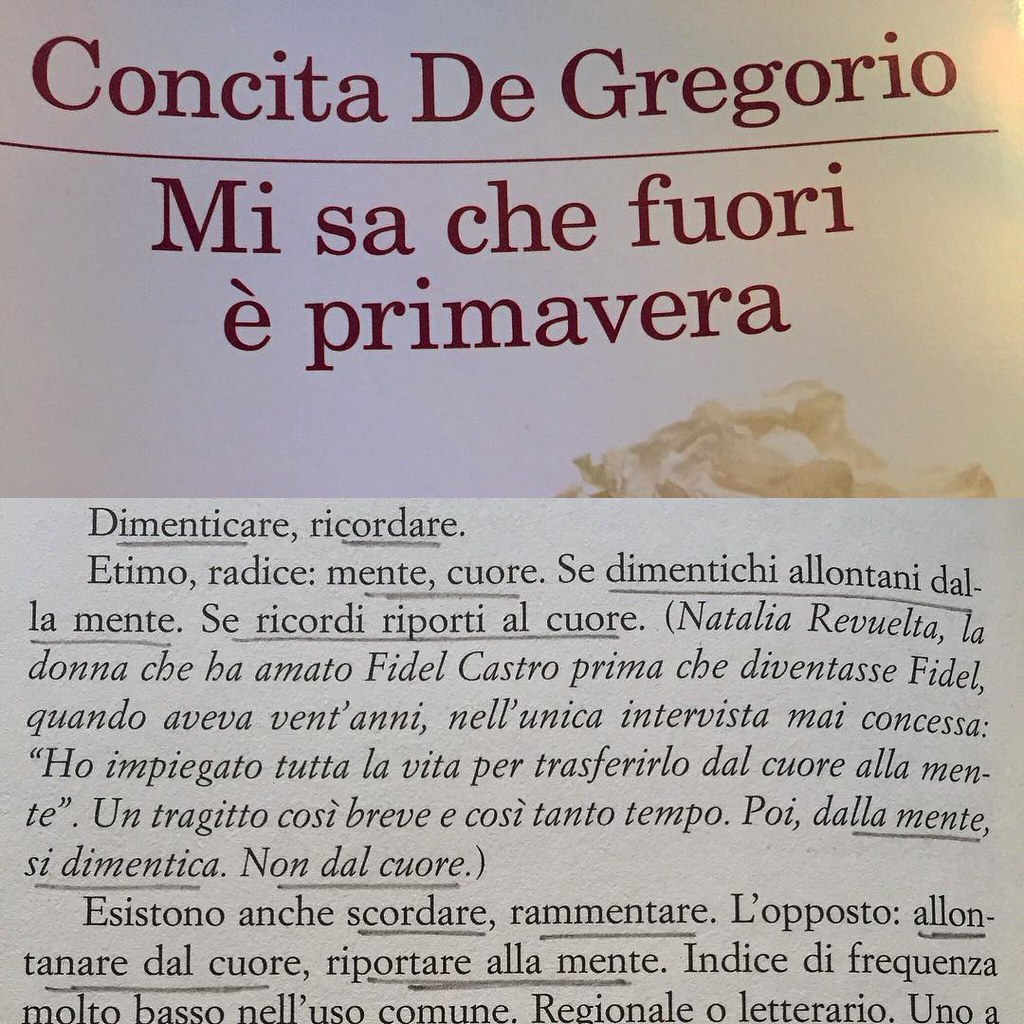The image depicts a piece of paper with text written in Italian, placed against a gray background that transitions from a darker shade at the top to a lighter shade at the bottom. The top section of the paper features burgundy letters spelling "Consita di Gregorio, Misa Cefiori e Primavera." Below this, in the lighter gray area, there are smaller black letters that read "Dimenticare ricordare attimo vatice mente cuore," with some additional text continuing further down. Several words throughout the document have been underlined in pencil, suggesting that someone has been taking notes directly on the paper.